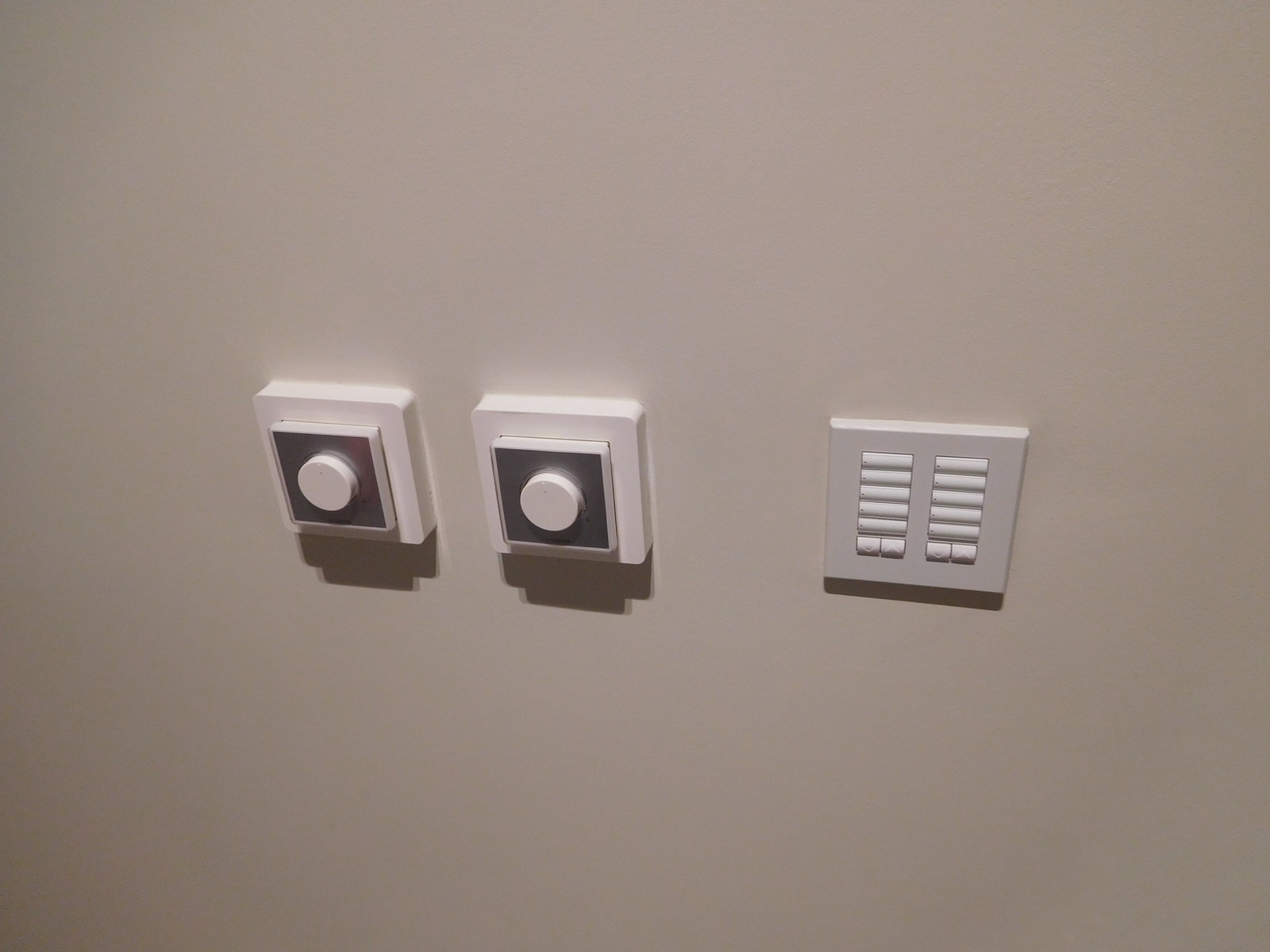A plain white wall, potentially situated in an office or an apartment block, features three distinct panels. The panel on the right resembles a complex doorbell system for multiple flats. Its appearance is somewhat out of place, as it is structured like a light switch socket but instead houses an array of rectangular buttons. There are two columns of buttons that look like small, stacked logs. This arrangement consists of five longer buttons at the top, followed by two thicker, shorter ones below, arranged in two columns. The exact function of these buttons remains unclear.

To the left of this panel are two push-button switches. These switches likely control lighting in this communal area, such as in a student dormitory. When pressed, they turn the light on but gradually release to turn the light off, aiding in electricity conservation. These two buttons are positioned side by side, though their precise purpose remains ambiguous.